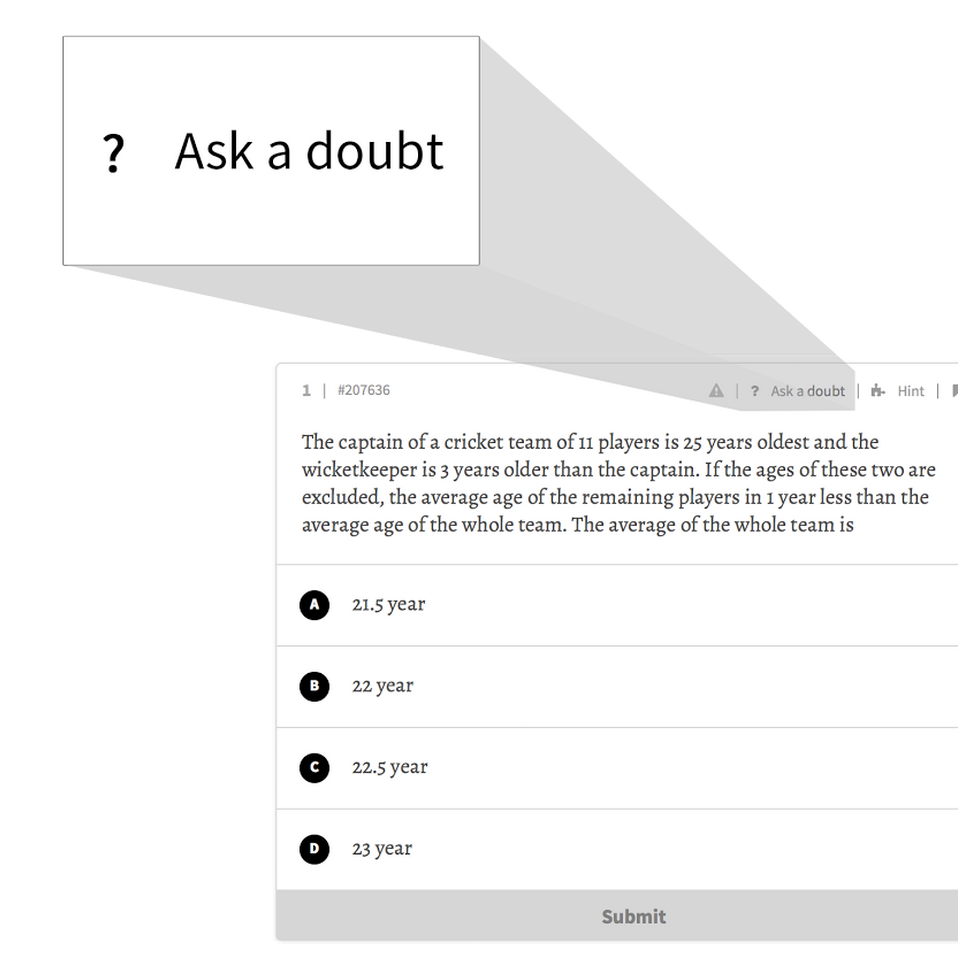In the top section of the image, there is a white rectangle outlined in black with a black question mark inside it. This section appears three-dimensional due to a shaded gray background, creating a shadow effect. Below the rectangle, the text "Acts with capital A, a doubt" appears. 

The main page depicted is cut off on the right side, but it includes a thin gray line running horizontally at the top, vertically down the left side, and horizontally across the bottom. The background is primarily white with gray accents.

In the top left corner, there is the text "1" followed by a vertical line, then the number "207636". On the opposite side, there is a gray triangle with a white exclamation point inside it. Below this, the phrase "The question mark acts, a doubt" is repeated. 

Further down, the text "Hint:" is followed by a detailed mathematical problem. The problem states: **"The captain of a cricket team of 11 players is 25 years old, and the wicketkeeper is three years older than the captain. If the ages of these two are excluded, the average age of the remaining players is one year less than the average age of the whole team."**

The problem then asks for the average age of the whole team, providing the following multiple-choice options:
- **A. 21.5 years** (displayed in white on a black circle)
- **B. 22 years** (displayed in white on a black circle)
- **C. 22.5 years** (displayed in white on a black circle)
- **D. 23 years** (displayed in white on a black circle)

At the bottom of the image, there is a gray rectangular box with a darker gray outline containing the word "Submit."

Ideal for making this descriptive caption vivid and comprehensive.